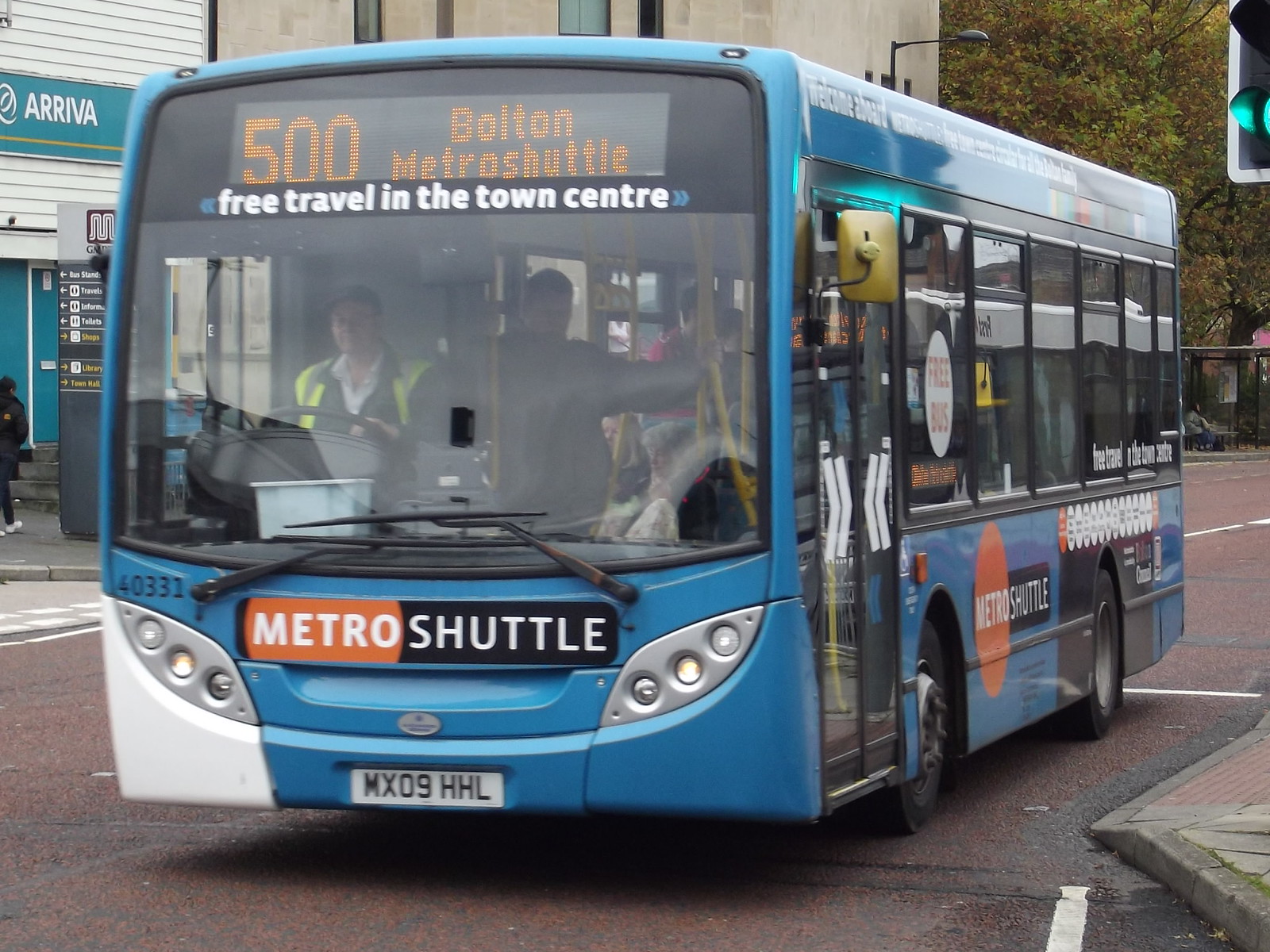A vibrant blue bus is seen traveling down a bustling city street. The bus, marked with "Metro Shuttle" underneath the windshield, offers free travel within the town center, as indicated by bold white lettering above the windshield. A digital display located at the very top of the bus announces its route as "500 Bolton Metro Shuttle Shuttle." Through the windshield, the bus driver is visible, clad in a distinctive black and yellow jacket. The side of the bus is similarly branded with the "Metro Shuttle" logo and adorned with several advertisements, adding a splash of color and information to the vehicle.